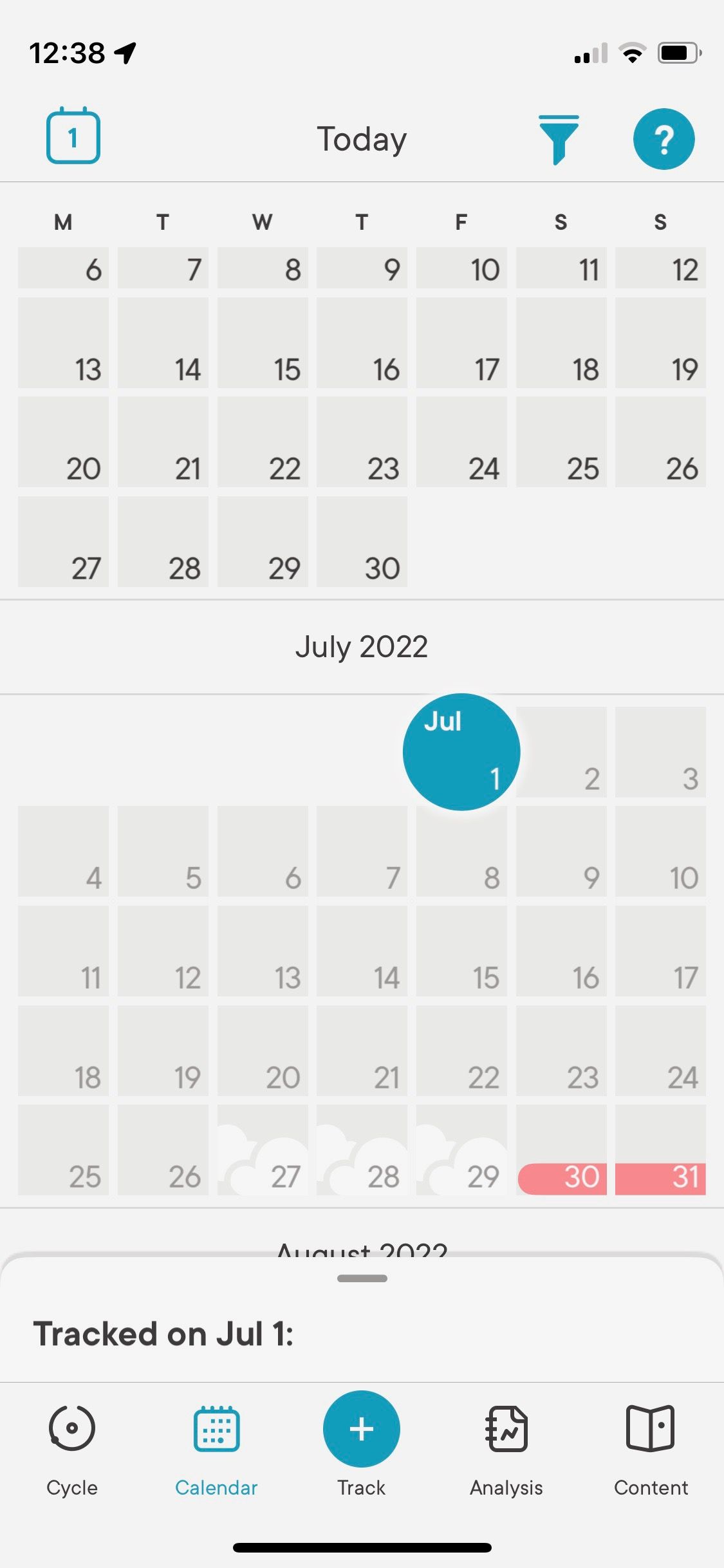**Detailed Screenshot Description:**

The screenshot captures the user interface of a period tracking app.

- **Top Bar Elements:**
  - **Time:** Displayed as "12:38".
  - **Paper Airplane Icon:** Located next to the time, possibly indicating a message or notification.
  - **Wi-Fi Signal:** Shows an active connection.
  - **Signal Strength:** Indicates cellular signal with two filled bars.
  - **Battery Icon:** Displays the battery status without a percentage indicator.
  
- **Main Screen Overview:**
  - **Background:** Predominantly gray with black font.
  - **Teal Calendar Icon:** Shows the number "1" inside it.
  - **Title:** "Today" is highlighted in black.
  - **Teal Funnel/Flashlight Icon:** A unique icon that looks like a combination of a funnel and a flashlight.
  - **Teal Question Mark Icon:** Enclosed in a teal circle, possibly for help or information.

- **Calendar Details:**
  - **Days Displayed:** Monday through Sunday.
  - **Dates Shown:** From the 6th to the 30th of the month, which appears to be July 2022.
  - **Highlighted Dates:**
    - **1st:** Marked with a teal circle.
    - **30th and 31st:** Highlighted in a reddish-pink color.
    - **27th, 28th, 29th:** Display cloud icons, perhaps indicating forecasted weather.

- **Additional Information:**
  - **Period Information:** Mention of "Tracked on July 1st".
  - **Cycle Tracking Elements:**
    - **Cycle:** A black circle calendar icon.
    - **Track:** A teal circle with a plus sign.
    - **Analysis:** A notebook icon with the letter "N".
    - **Content:** Represented by a book icon.

- **Navigation Bar:**
  - Details appear to blur into a black bar at the bottom, indicating potentially hidden or navigational elements.

- **Context Clues:**
  - The partial calendar view above likely represents June, transitioning into a full view of July.

Overall, the image represents a detailed interface of a period tracking application, complete with calendar details, tracking features, and navigational icons.